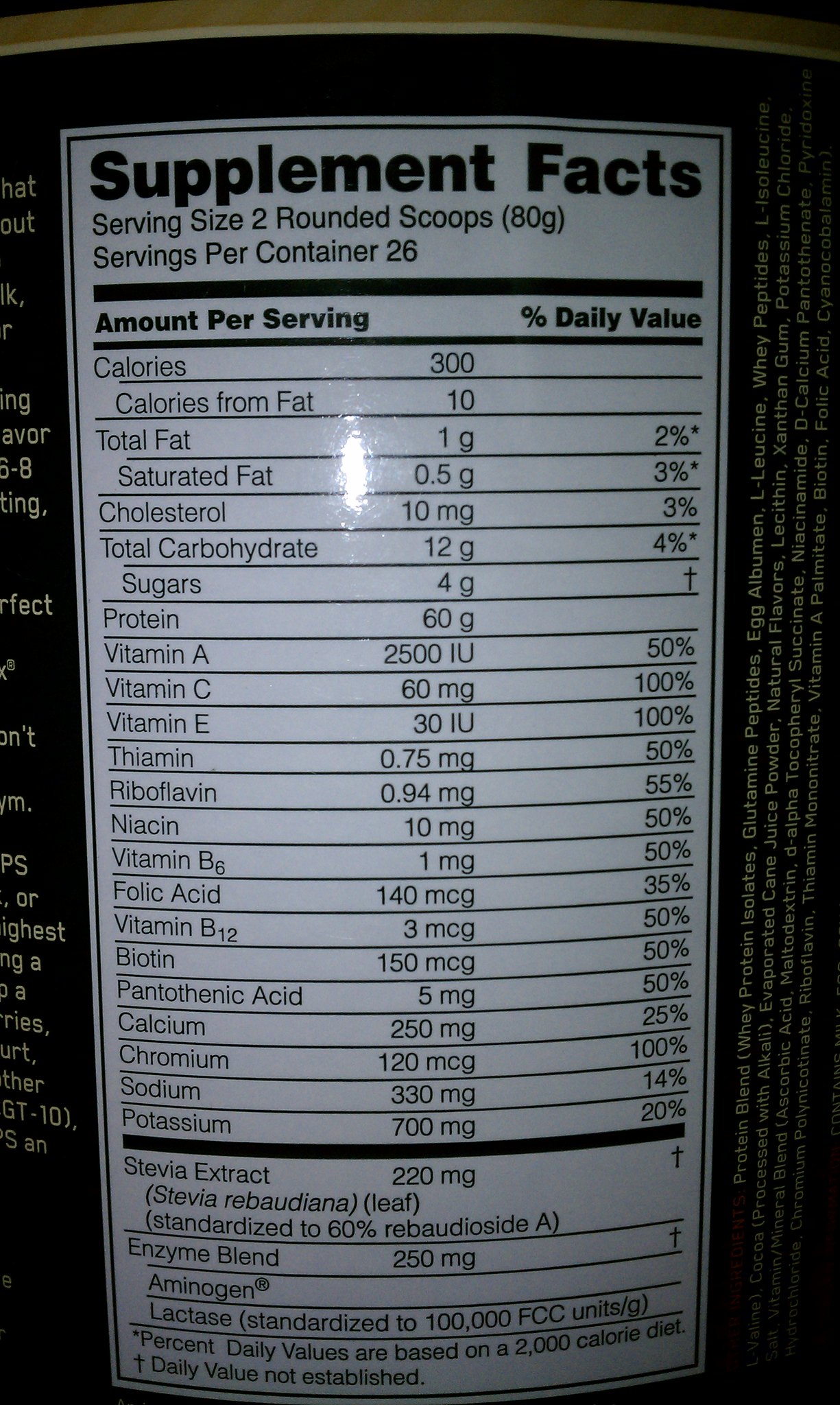The image is a photograph of the nutrition label from a supplement canister. The label, predominantly a white rectangle, features black text detailing the supplement facts. At the top of the label, the heading "Supplement Facts" is prominently displayed in bold black lettering. Below this heading, the label provides comprehensive nutritional information, listing various vitamins and minerals. It specifies that the serving size is two rounded scoops, with a total of 26 servings per container.

The label includes numerous details in black font, offering a thorough breakdown of the supplement's nutritional content. The background of the label subtly blends into the rest of the canister, which is characterized by a dark, likely black, color adorned with white text. The canister is topped with a gold-colored lid, adding a touch of elegance to the overall appearance.